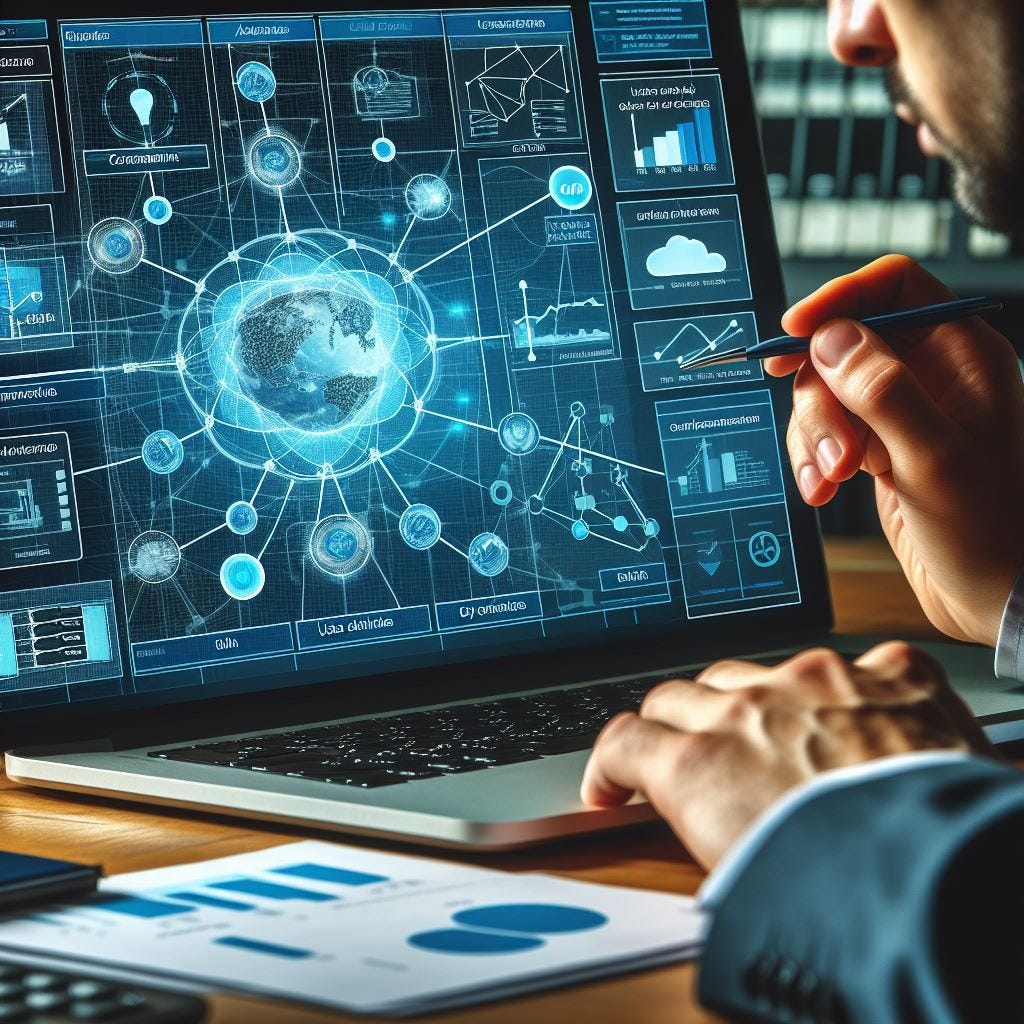The photograph captures a close-up view of a man, likely Caucasian, intently examining a laptop screen filled with complex data. His dark facial hair and parts of his face, including his nose and mouth, are partially visible. The man is dressed in a suit, suggesting a professional environment. His left hand rests on the silver keyboard of the laptop, which features black keys, while his right hand, holding a stylus or pen, points towards the screen. The screen displays a dark interface dominated by blue elements, showcasing a detailed diagram resembling a globe with lines and smaller circles radiating from it, alongside numerous graphs in squares on either side. Although the exact text on the screen is unreadable, it seems to present a scientific problem or demonstration. The laptop is placed on a brown desk, surrounded by various items, including white papers with blue graphs and a possibly blurred calculator in the corner. Additional indistinct objects are visible in the background near the man's face, adding depth to the scene.